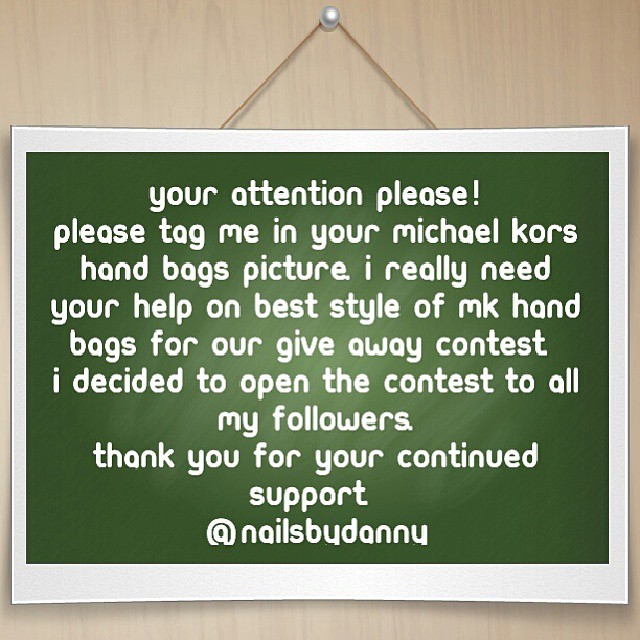The image features a square banner hanging from a tan surface, secured by a string tied to a nail positioned at the top center of the image. The banner has a white border and a dark green background with white, lowercase text. The text on the banner reads: "your attention please! please tag me in your Michael Kors handbags picture. I really need your help on best style of MK handbags for our giveaway contest. I decided to open the contest to all my followers thank you for your continued support - @NailsByDanny." The color palette of the image includes shades of tan, silver, brown, white, and green. This appears to be a digital creation, likely intended for sharing on social media platforms.